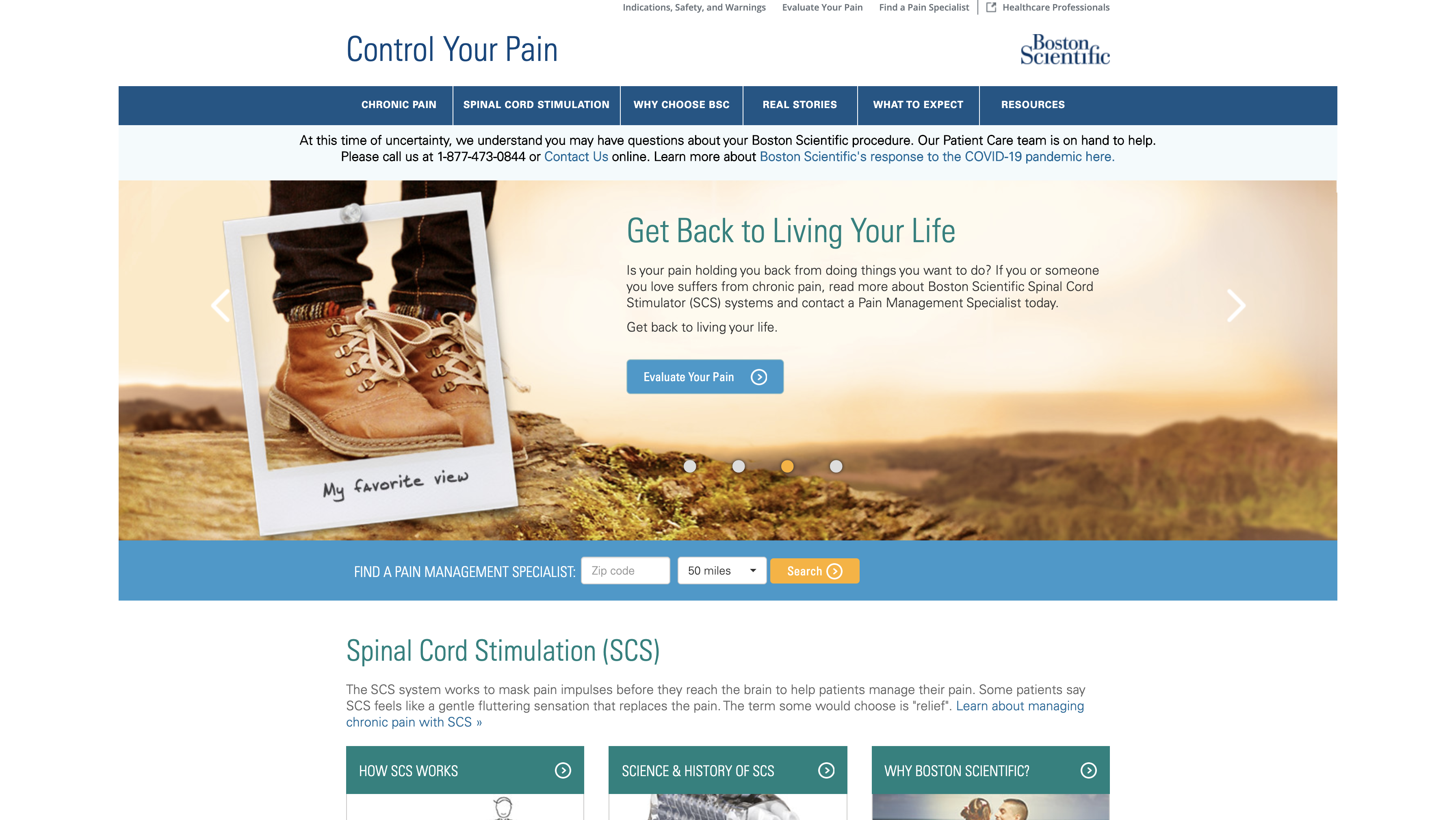This screenshot captures the homepage of Boston Scientific's website, specifically designed to help users manage pain. Prominently featured, the Boston Scientific logo is positioned at the top right, while a striking headline "Control Your Pain" occupies the top left. Dominating the page is an evocative main image depicting an expansive canyon with oversized feet and legs, complemented by the encouraging headline "Get Back to Living Your Life." Below the image, there is insightful text copy and a prominent blue button labeled "Evaluate Your Plan."

The top of the page features a blue menu bar offering several navigation options: Chronic Pain, Spinal Cord Stimulation, Why Choose BSC, Real Stories, What to Expect, and Resources. Beneath this bar is a brief note addressing COVID-19-related concerns. Additionally, a blue rectangular banner invites users to "Find a Management Specialist," allowing them to input their zip code and begin a search.

Although the screenshot does not capture the entire homepage, it reveals that the next section is dedicated to spinal cord stimulation. This section includes three informative videos and additional text copy for users to explore. Overall, this screenshot provides a comprehensive overview of the initial segments of Boston Scientific’s homepage, geared towards guiding users in pain management.